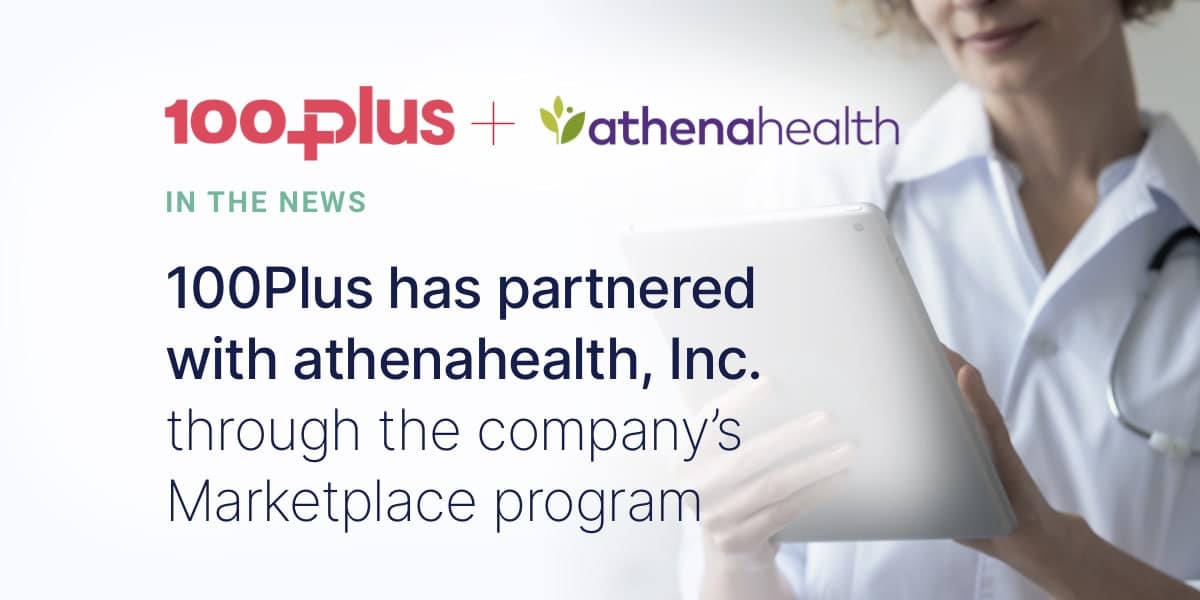This image is a digital advertisement for Aetna Health, captured as displayed on a computer screen. The advertisement features a predominantly white background that gradually transitions into an image of a healthcare professional, likely a doctor or nurse. The focal point is a white woman with short brown hair, adorned in a white lab coat. Visible around her neck is a stethoscope, and she is holding a tablet elevated in front of her.

Prominently written in red text at the top of the advertisement is "100+," followed by a green plus symbol adorned with multicolored leaves, leading into the Aetna Health logo. Directly below this, in green text, reads "In the News."

The primary message of the advertisement is emphasized in bold black text: "100+ has partnered with Aetna Health Inc." Below this statement, in standard black text, it mentions that this collaboration is conducted "through the company's marketplace program."